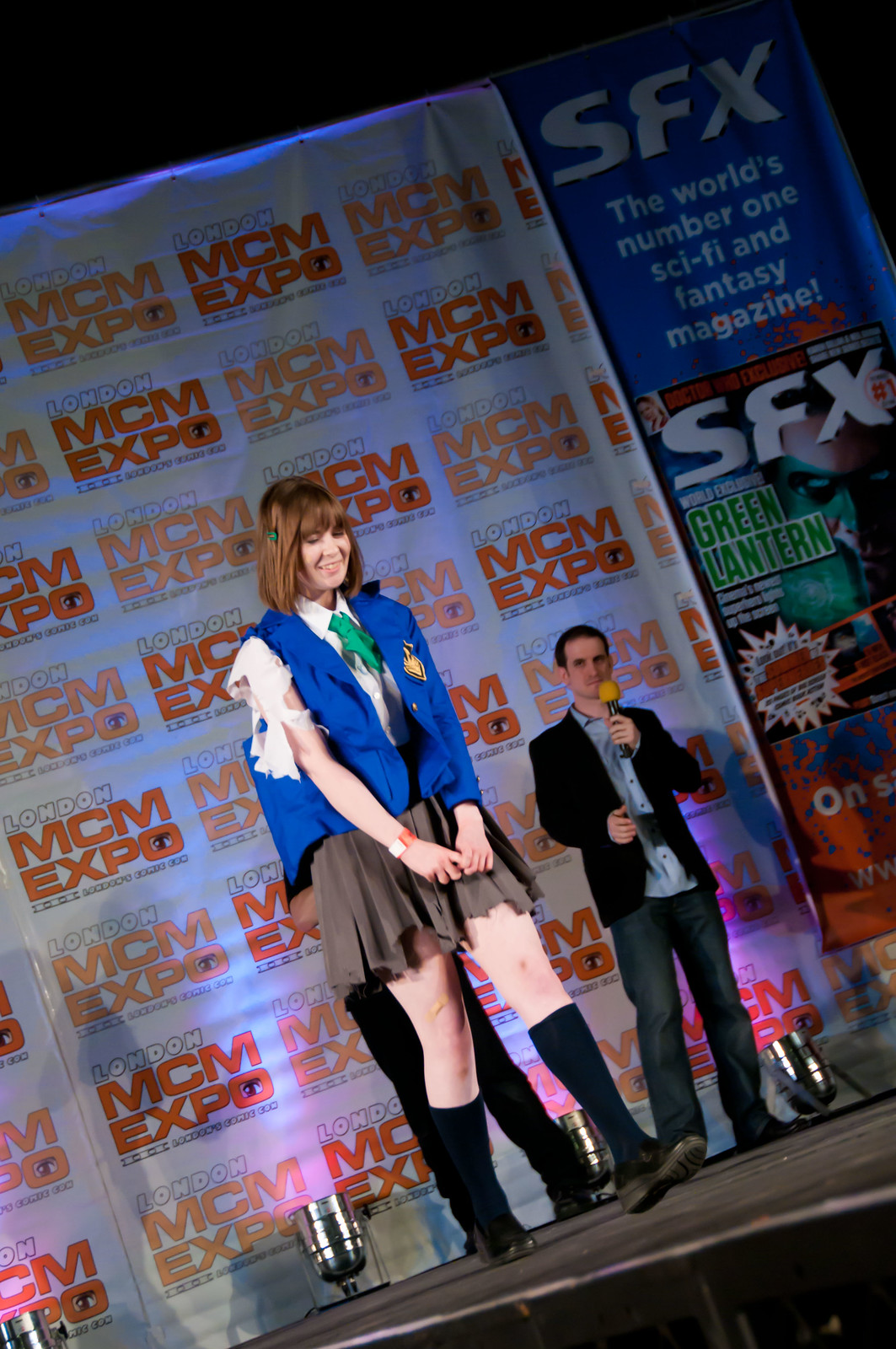In the forefront of this image, a young woman, possibly in her 20s, commands attention at what appears to be an exposition, likely the London MCM Expo, as indicated by the repeating signage in the background. She has distinct brown hair with bangs and wears a somewhat eclectic ensemble: a white button-up shirt that's notably shredded, a green tie, a blue vest or jacket, a brown rippled skirt, and black knee-high stockings paired with black shoes. Despite her downward, bashful gaze, she smiles serenely.

Dominating the backdrop, a large sign prominently reads "London MCM Expo" in varying shades of orange and white, set against a predominantly black background. Additional signage on the right side proclaims "SFX The World's Number One Sci-Fi and Fantasy Magazine" with an image of a magazine featuring the "Green Lantern." 

Behind the woman, to her side, a white man, appearing to be in his late 20s to early 30s, sits holding a microphone. He dons a blue button-down shirt, a blazer, and jeans. Another pair of legs, suggesting the presence of another person partially obscured by the woman, is also visible in the scene. Overall, the vibrant scene appears to capture a candid moment of an exposition, with both central figures poised amid a sea of geeky festivities.